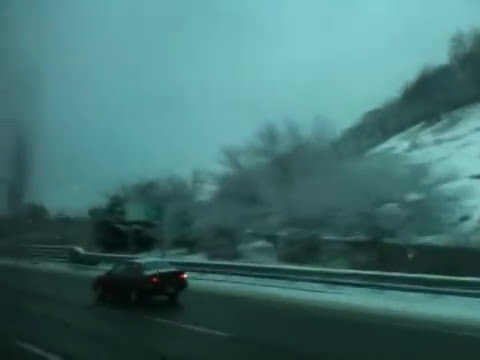The image captures a winter scene on a high-speed highway, likely taken during the daytime. The main focus is a car in motion, traveling towards the left of the frame with its red taillights visible through a haze that suggests snow might be falling, impacting the photo's clarity. The vehicle and the multi-lane road are both dusted with snow, indicating recent snowfall. On the right side of the road, there is a guardrail and possibly a small fence that runs alongside a snow-covered hillside, which is topped with sparse trees and a large bush at the center. In the background, additional details like a small shed or house can be faintly seen near the fence. The overall color palette is dominated by whites, blacks, various shades of grey, and the striking red of the taillights, emphasizing the wintry outdoor setting.